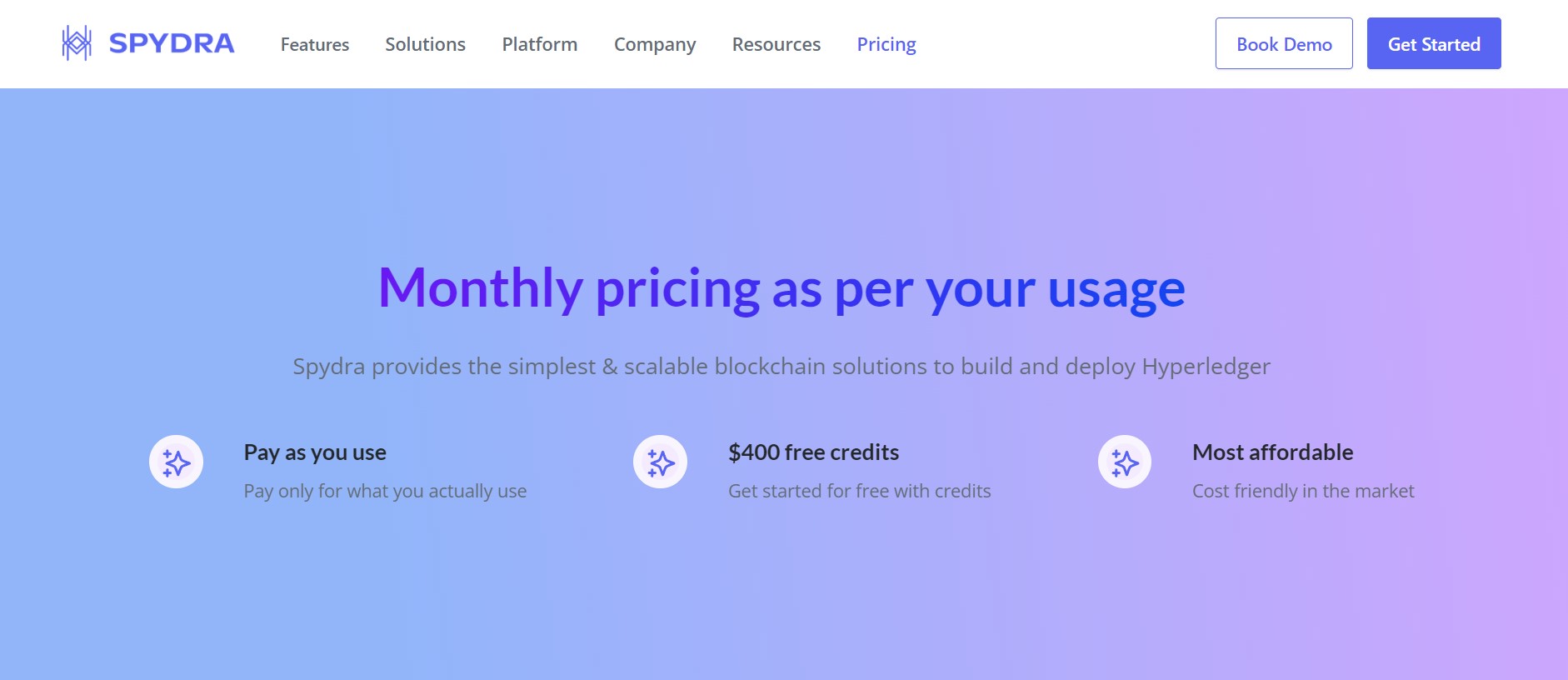"Introducing Spydra: A minimalistic and modern graphic representation of a spider, cleverly designed using general shapes. At the center, a prominent diamond shape is flanked by pseudo-leg extensions. Overlaying the spider graphic are links to various sections including Features, Solutions, Platform, Company, Resources, Pricing, with buttons to 'Book Demo' and 'Get Started' prominently displayed. The visual palette transitions from blue to purple, adding a sleek and professional touch. Additionally, Spydra emphasizes a pay-as-you-use model offering scalable blockchain solutions tailored for Hyperledger projects. With benefits such as $400 free credits and affordability, Spydra promises the simplest way to build and deploy blockchain applications."